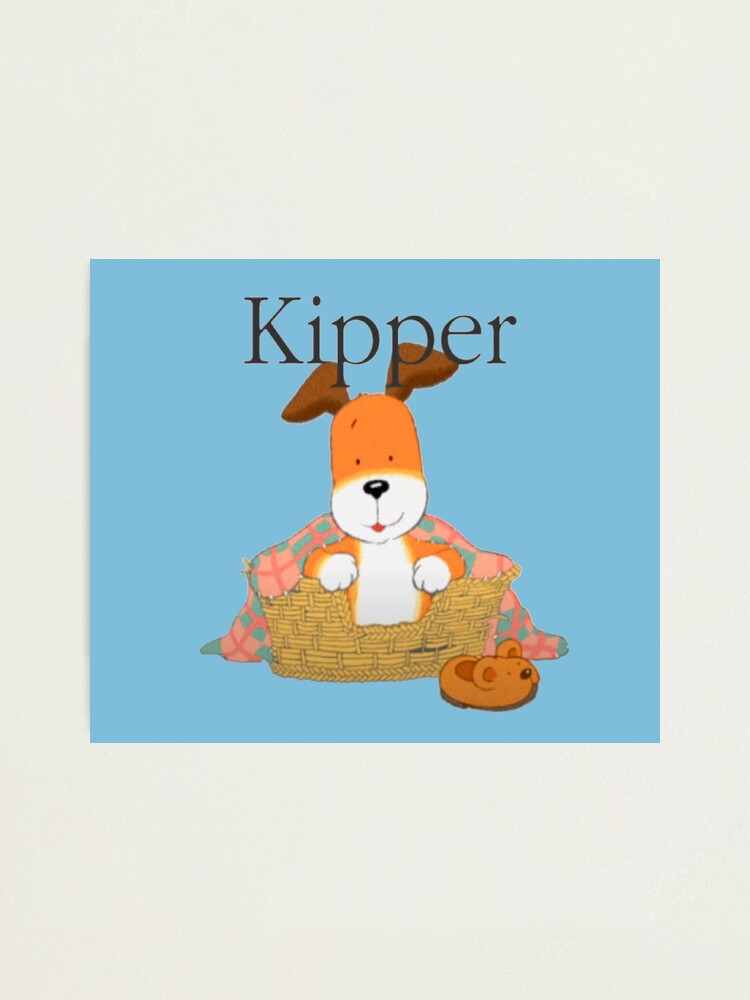This is a vibrant, juvenile-style illustration of a smiling dog sitting inside an oval-shaped wicker basket that seems to double as a cozy dog bed. The basket features a small front opening and is wrapped in a pink and green checked blanket that drapes over its edges. The dog, named Kipper as indicated by the black "Times New Roman" style text above his head, has a cheerful expression with his red tongue playfully sticking out. He has a brown coat with white markings on his face, chest, paws, and underbelly. His distinct brown ears stick up, pointing in opposite directions. The composition is set against a light blue background with a small brown slipper, resembling either a bear's or mouse’s head, placed in the bottom right corner. This detailed and whimsical cartoon drawing captures a moment of warmth and friendliness, making it appealing and endearing.